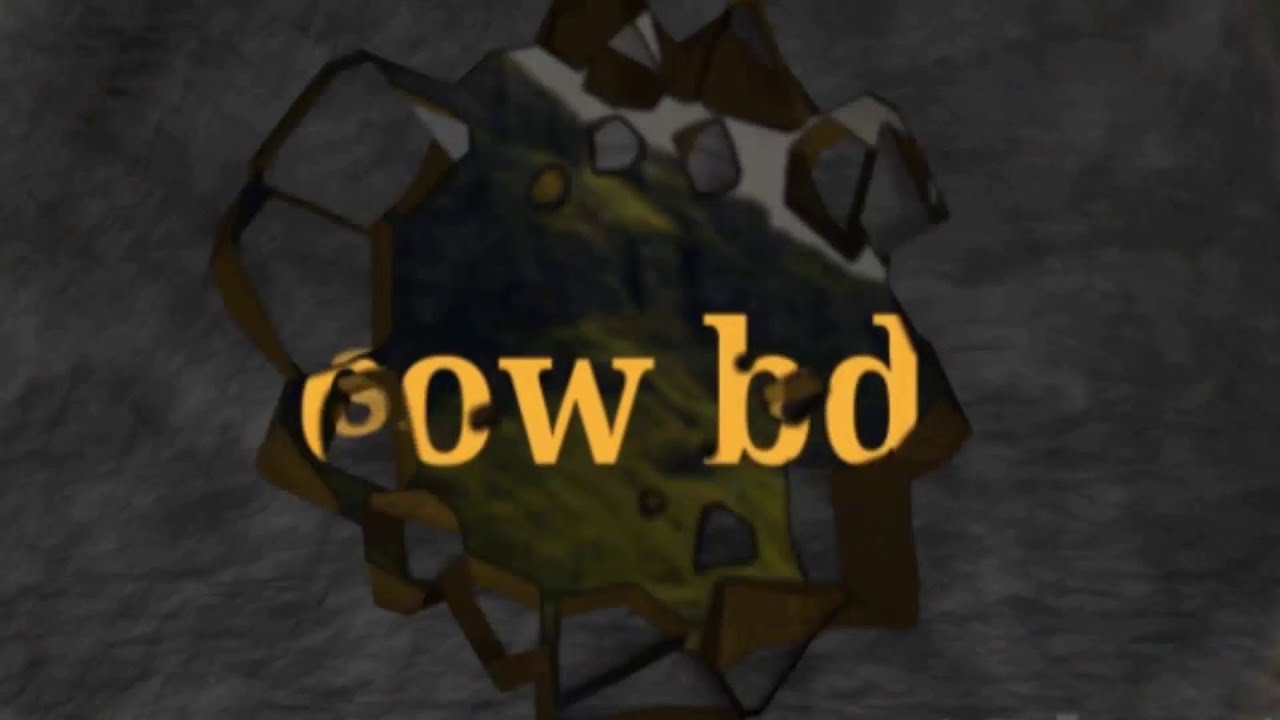The image showcases an artist's creation that appears to be a mixed-media piece, possibly a painting, chalk drawing, or marker work, enveloped in a shadowy, textured background of grays and blacks. The central composition features a complex geometric formation with various shapes, resembling a crumpled paper or meteorite. This centerpiece combines hues of moss green, black, and coppery brown, with gaps revealing the backdrop. The background gives a smudgy, striped feel, enhancing the overall gloomy and dark atmosphere. At the core, the geometric rock figure includes shapes like triangles, rectangles, and near-circles, presenting a diverse conglomerate effect. The entire piece exudes a low-resolution, soft-focus aesthetic, reminiscent of early CGI or video game cutscenes, with a stone wall-like texture kissed by overcast skies. Overlaid in a distressed manner across the rock are fragmentary letters "S O W   B D" in a gold or yellow hue, some obscured by the shapes, lending an aged, mysterious charm to the artwork.